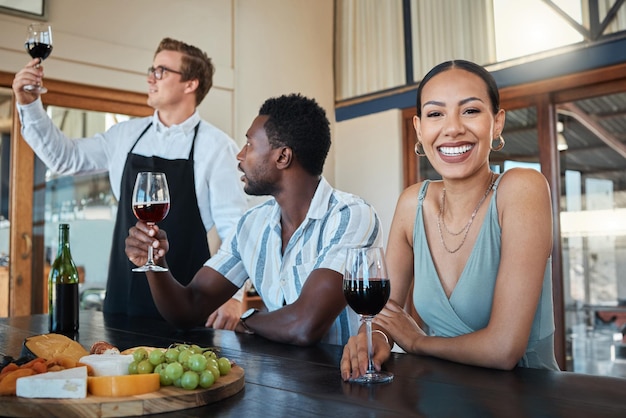In this indoor, daytime photograph, three people are gathered at a wine tasting event, seated around a dark brown hardwood table adorned with a charcuterie board featuring grapes, cheeses, and possibly other fruits or meats. To the right, a smiling Hispanic woman in a light blue dress is looking directly at the camera, her hoop earrings and necklace adding to her cheerful appearance. To her left, a Black man with close-cropped hair is sitting with his elbows on the table, raising a glass of wine, absorbed in conversation as he looks at another man. This third individual, a white man with dirty blonde hair and plastic glasses, is dressed in a white shirt and black apron, inspecting a glass of wine. This figure, likely an employee of the restaurant, carefully examines the wine, adding a touch of professional inquiry to the scene. Behind them, light streams in through a glass door and a window above, further illuminating the cozy atmosphere of this wine tasting.